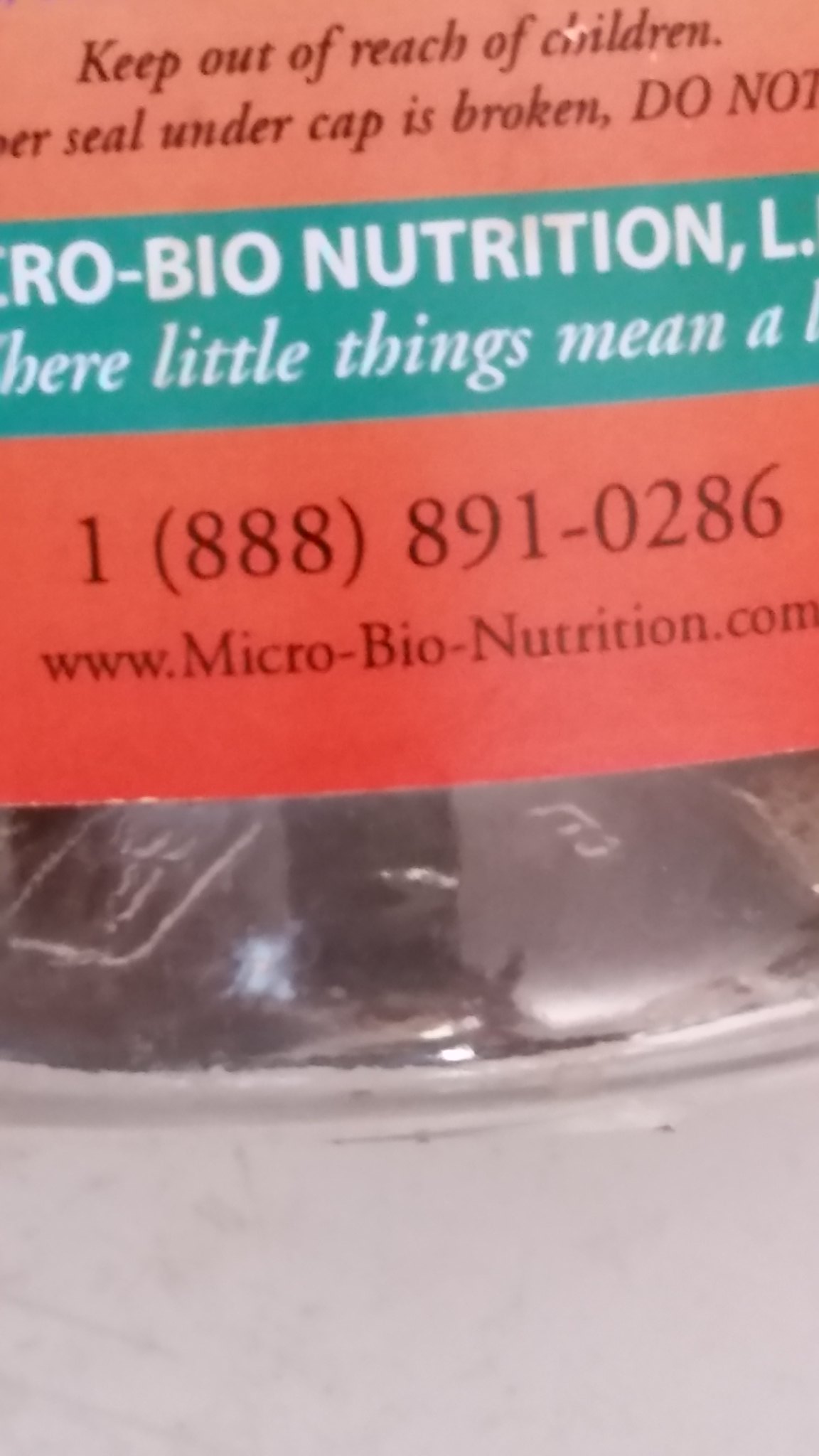This close-up image captures the lower portion of a bottle, possibly made of glass or plastic, containing a clear liquid. The bottle appears to be a product related to bio-nutrition. The label, which is predominantly green, features the brand name "Bio-Nutrition" in white lettering, along with the slogan "Where Little Things Mean a Lot." Above this main label, a warning advises to "Keep out of reach of children." Below the green label, there is a section that includes a toll-free number and a URL for the manufacturer's website, offering ways to contact the company. The bottle is placed on a white surface, emphasizing its clarity and the detailed labeling.